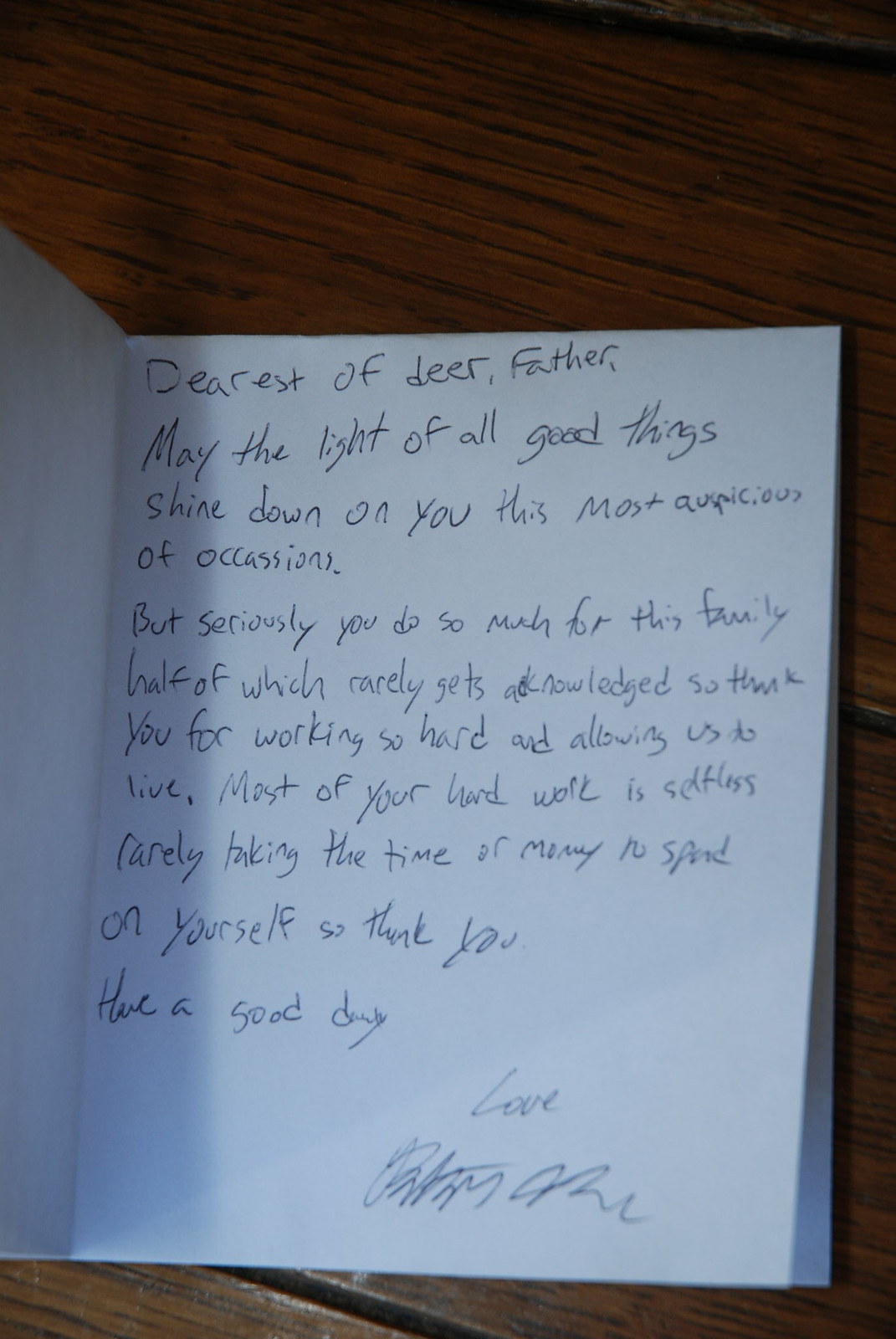This image captures a close-up of a greeting card, likely received through the mail for a special occasion such as a birthday, resting open on a dark brown wooden desk or table with visible wood grain. The card, which appears to be homemade, features a heartfelt handwritten message in black ink on a white background. The message reads: “Dearest of dear father, may the light of all good things shine down on you this most auspicious of occasions. But seriously, you do so much for this family, half of which rarely gets acknowledged. So thank you for working so hard and allowing us to live. Most of your hard work is selfless, rarely taking the time or money to spend on yourself. So thank you. Have a good day. Love,” followed by an unreadable handwritten signature. The scene conveys a touching and personal expression of gratitude and love.